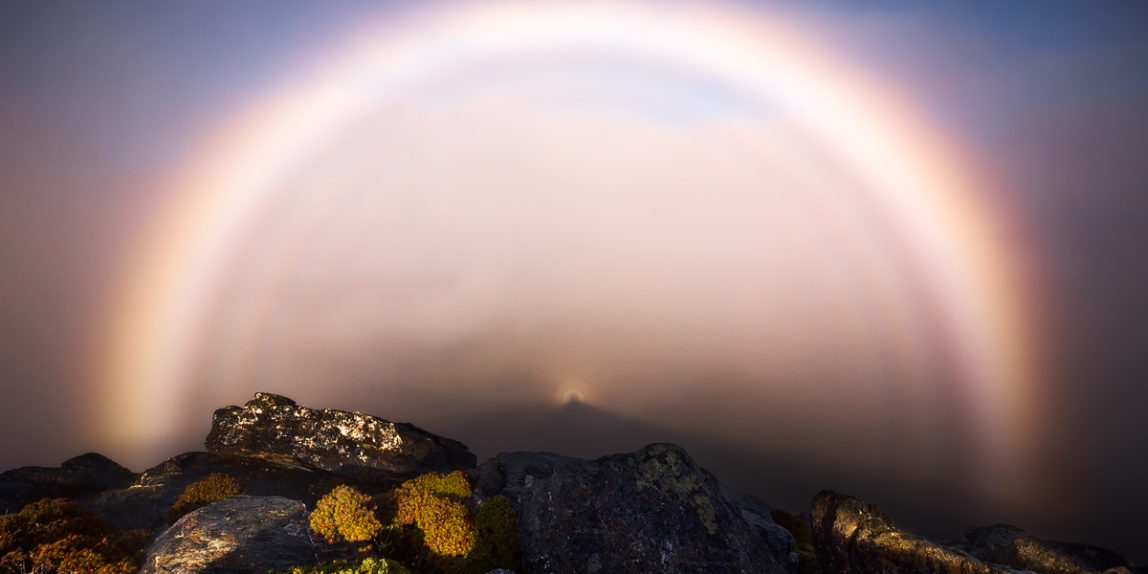The image captures a surreal and futuristic natural landscape, appearing to be taken from a mountaintop. Dominating the scene is a blurred, arc-shaped bright light resembling a rainbow but in shades of white and yellow, creating an almost mystical or otherworldly feel. This blurred light formation gives the illusion of looking into a distant tunnel amidst a backdrop of a blue sky. The foreground is lined with various rocks, primarily dark brown with some appearing bluish or black with white speckles. Interspersed among the rocks is a cluster of green trees, adding a touch of vibrant life to the rugged terrain. Notably, the rocks show intricate details, such as hints of moss or dirt. The overall composition combines an ethereal light display with the stark solidity of nature's elements, producing a uniquely abstract yet beautifully natural scene.